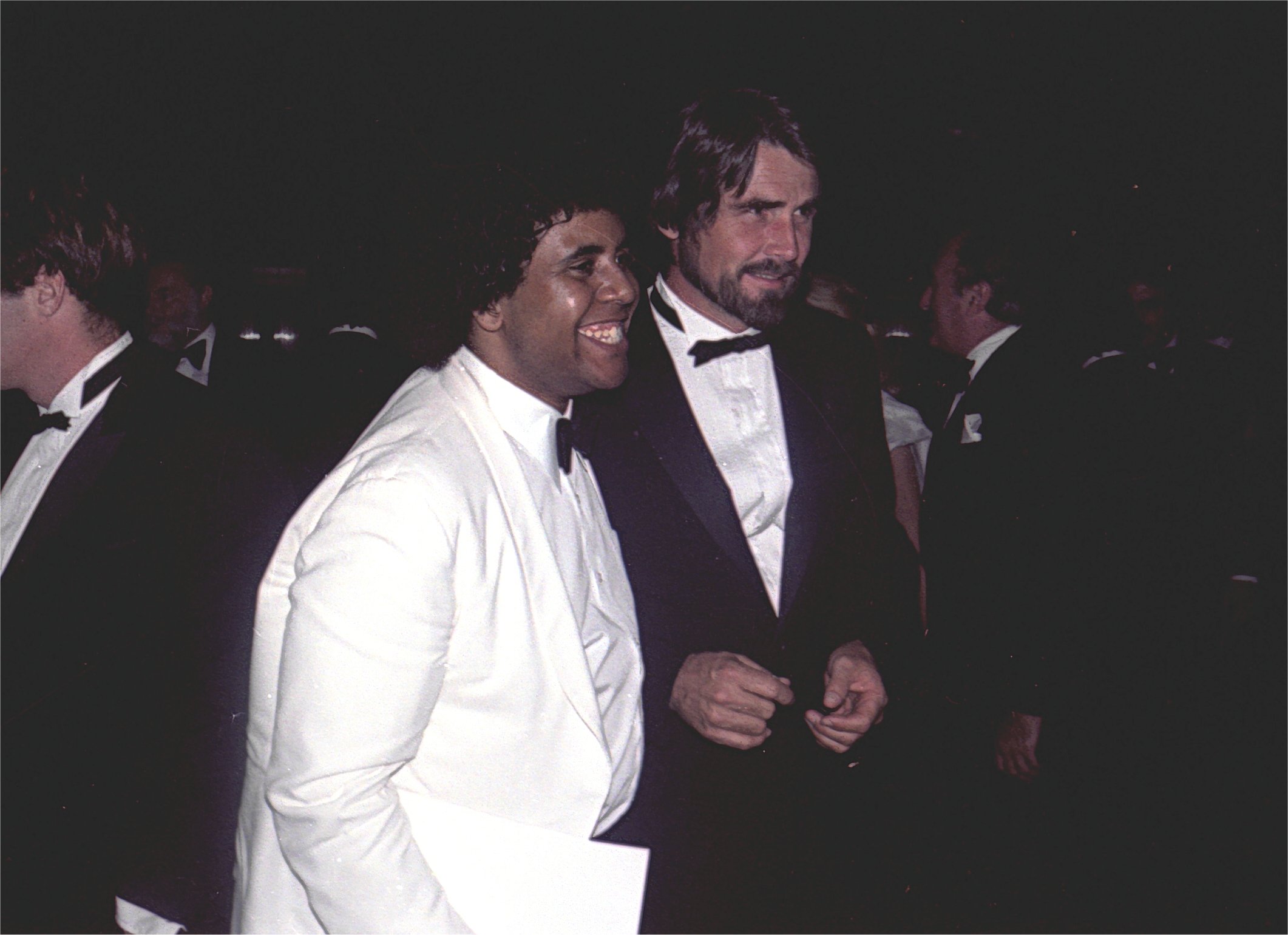In this dimly lit, crowded scene of a formal event, the photograph showcases two men prominently in the foreground, surrounded by other indistinguishable figures in the shadowy background. The man on the left, with darker skin and black curly hair, is smiling as he faces towards the right. He is dressed in a white dress jacket paired with a white dress shirt and a black bow tie. Beside him, to the right, stands a lighter-skinned man with a neatly groomed beard and mustache. He also faces towards the right, clad in a black dress jacket, white dress shirt, and a matching black bow tie. His hands are held at waist level in front of him. The background reveals faint outlines of more people dressed in formal attire, all enveloped in near darkness that creates an impression of a black void, lightly hinting at the possibility of an outdoor setting with obscured buildings.